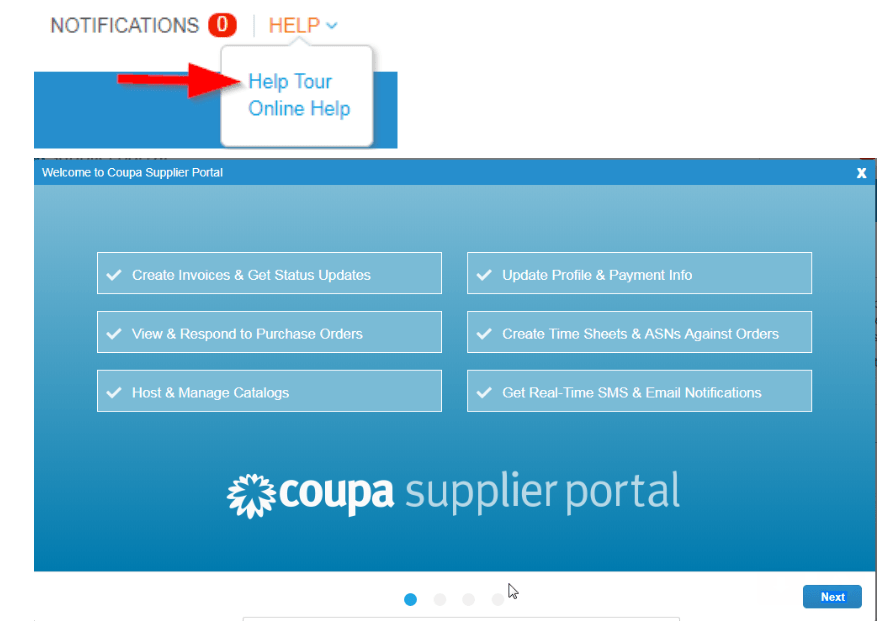The screenshot features the Coupa Supplier Portal interface, highlighted by several distinct elements. At the top of the screen, a notification bar is visible, which contains a 'Help' button that has been clicked. Activating this button has triggered a dropdown 'Help Tour' menu, also labeled 'Online Help', underscored by a digitally added red arrow for emphasis. Situated behind this dropdown is a blue rectangle, part of the portal's layout, which extends toward the bottom of the screen to a larger blue rectangle area. The top section prominently displays a "Welcome to Coupa Supplier Portal" message. To the far right of the top rectangle, an 'X' button offers the option to close this message. 

Further down, the bottom section of the screen reiterates "Coupa Supplier Portal" in white text paired with a decorative icon. In the bottom right corner, a blue 'Next' button stands out, designed for user interaction, with white lettering. Central to the interface, six checkable areas are arranged for navigation or selection purposes, providing users with actionable options within the middle section of the screen.